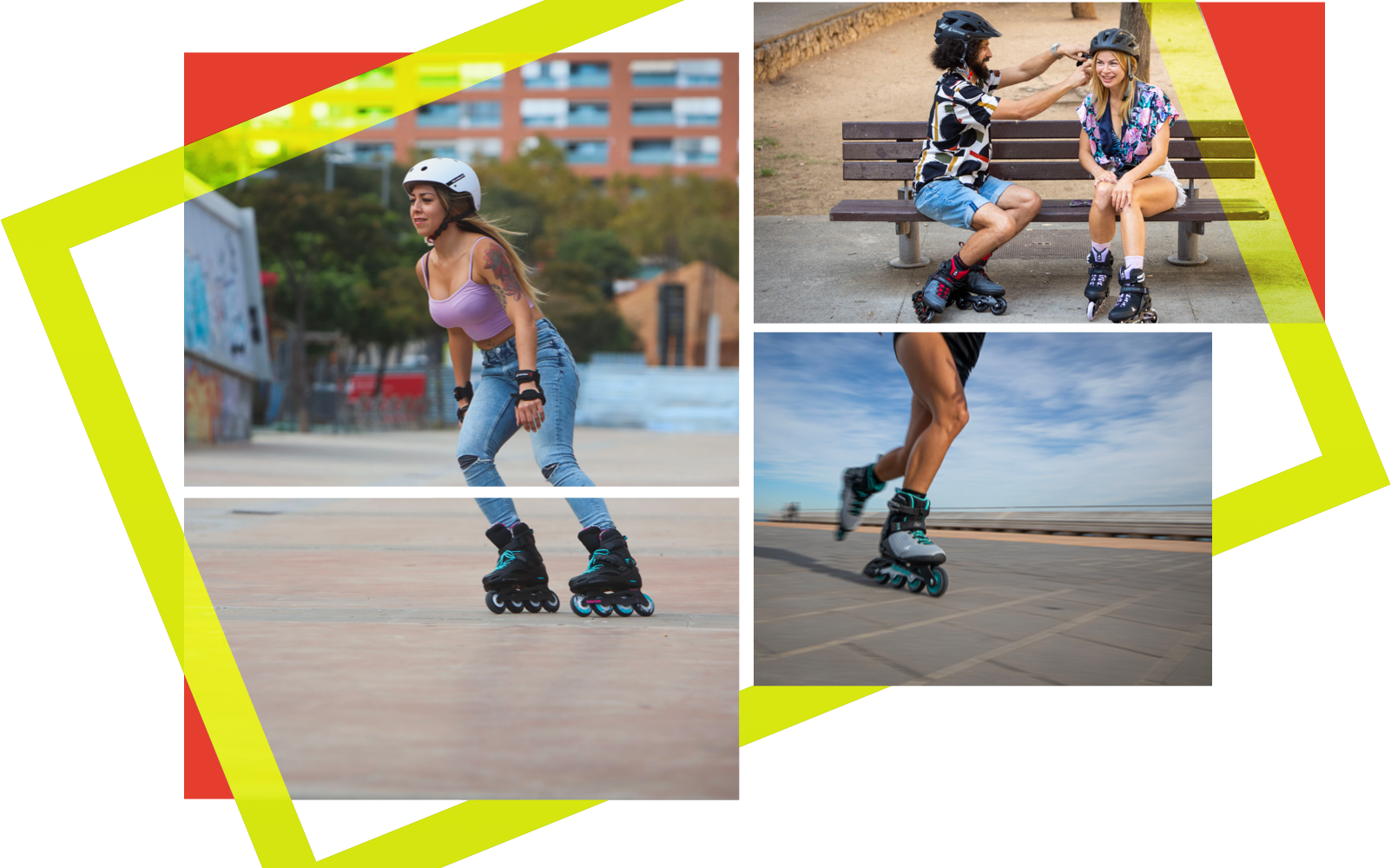This promotional image for rollerblading features a distinct Art Deco style and is framed by a diagonal yellow rectangular border with red accents in the corners. The image is divided into four rectangular sections, each highlighting various scenes of people enjoying rollerblading.

In the leftmost section, split into two parts, a woman with long, light brown hair and a tattoo on her left arm is shown rollerblading. She is dressed in a lavender tank top, blue jeans with holes at the knees, and wrist pads. Her rollerblades are dark blue with teal accents and hints of pink. She also wears a white helmet and a black watch. The background reveals a skate park-like area with a graffitied wall, numerous windows of nearby buildings, pavement, and some trees.

The top right section depicts a man and a woman sitting on a brown bench, both outfitted with rollerblades and black helmets. The man, with long hair, a beard, and a patterned shirt featuring white, red, yellow, and black colors, is helping the woman adjust her helmet. She has blonde hair, a colorful floral shirt, and short shorts. Her rollerblades are lavender and black, while his are gray with red accents. They sit on an asphalt sidewalk, with dirt visible in the background.

The bottom right section is a close-up of someone rollerblading, capturing the motion through a blur effect. The rollerblades are light gray and dark blue with teal, and the rollerblader has very tan, muscular legs. A beautiful day is indicated by the clear blue sky and scattered clouds in the background, which appears to be a beach scene.

This image beautifully captures the spirit and joy of rollerblading, making it an inviting promotional piece.